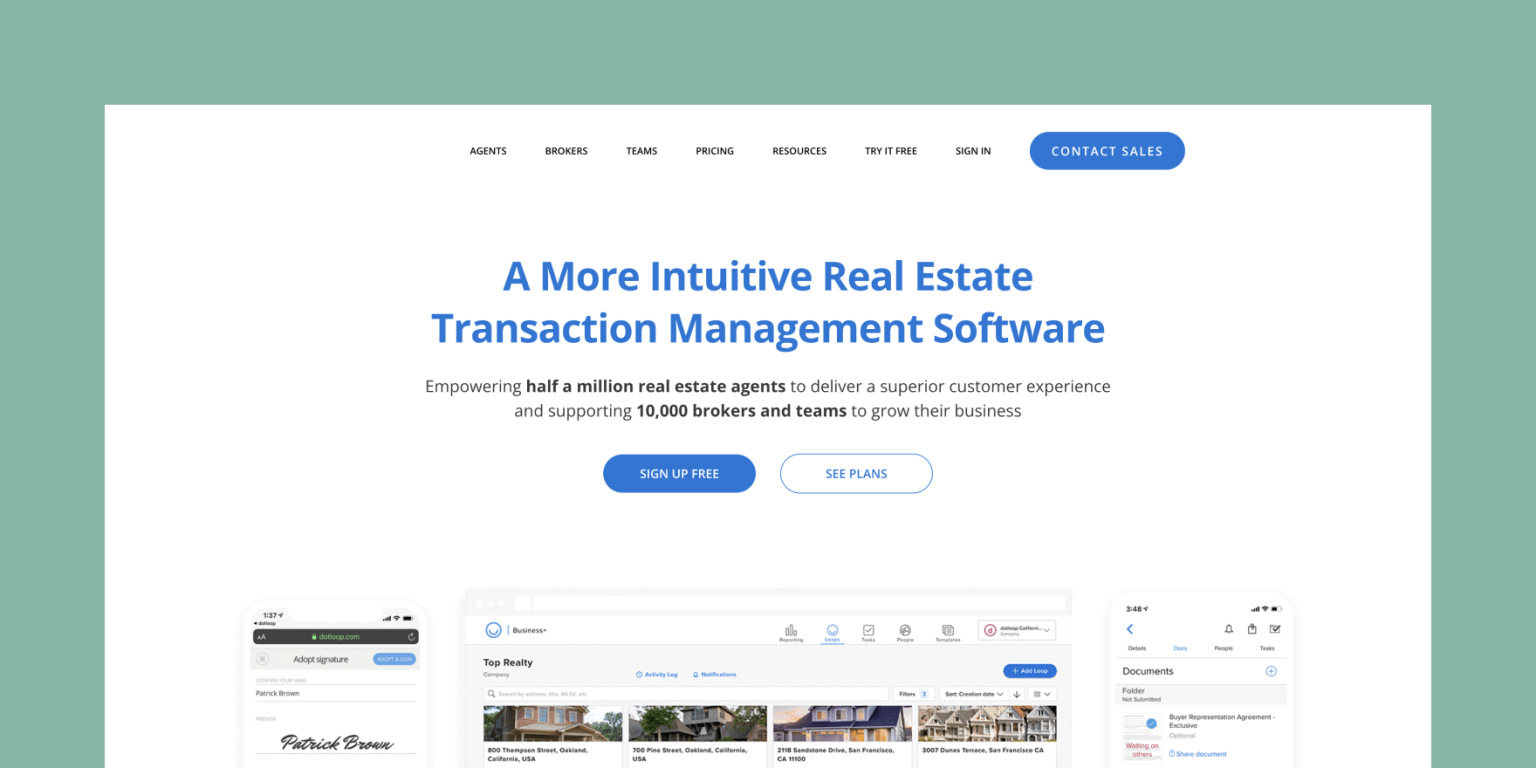The image depicts the homepage of a real estate website, framed by a thick aqua green border encompassing the top and sides of the webpage. The webpage appears cut off, displaying approximately half of its content. 

At the top of the webpage, various navigation options are listed, including "Agents," "Brokers," "Teams," "Pricing," "Resources," "Try it Free," "Sign In," with a prominent blue oval button labeled "Contact Sales."

Centered on the page, a headline reads "A More Intuitive Real Estate," followed by a subheading stating "Transaction Management Software." Further down, text emphasizes, "Empowering half a million real estate agents to deliver a superior customer experience and supporting 10,000 brokers and teams to grow their business."

Beneath this, two buttons are visible: a blue oval button labeled "Sign Up for Free" and a clear oval button labeled "See Plans."

The lower section of the webpage displays part of another segment featuring four images of homes, each separated into individual images. To the left, within a box, the word "Patrick" is displayed, alongside what appears to be an image of a phone. On the right side, another section of the phone image is visible, with the word "Documents" inscribed.